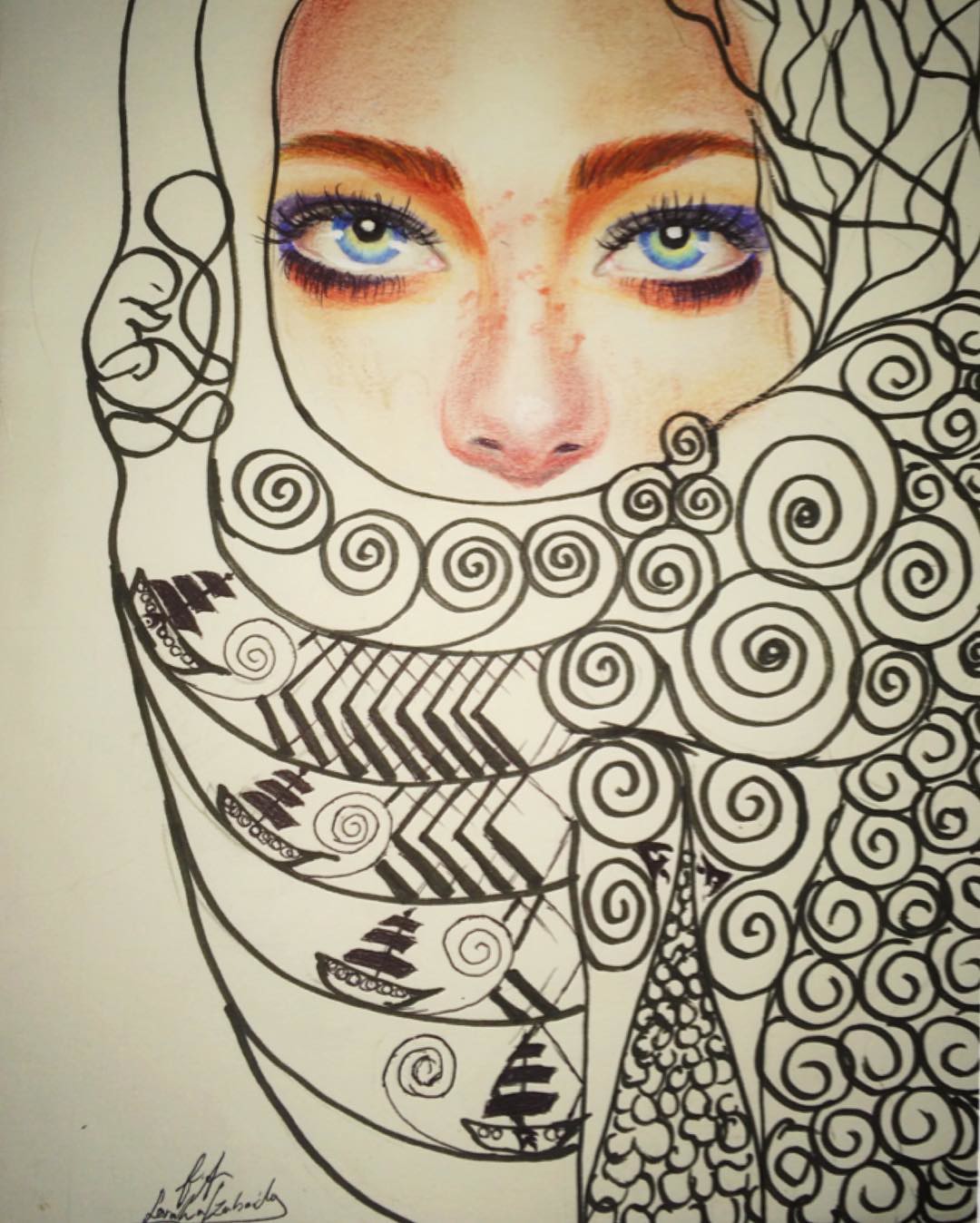This artwork features a light-skinned girl with blue eyes and freckles delicately sprinkled across her nose. Her eyebrows are rendered in a reddish hue, adding a contrasting warmth to her complexion. The girl gazes directly at the viewer, creating an intimate and captivating connection. The portrayal of her face, particularly the visible portions, is meticulously crafted with what appears to be colored pencils, showcasing realistic detail and subtle shading.

Her head and face are partially obscured by an elaborate headscarf that envelops her entire head and cascades down her body. This headscarf is distinctly different in style, drawn using bold, black marker outlines that form intricate squiggles, adding a textured and dynamic element to the composition. Interspersed within the squiggles are various ship-themed imagery, providing an additional layer of narrative and interest.

In the upper left-hand corner of the artwork, there seems to be a representation of a baby, adding further depth and perhaps hinting at a storytelling aspect within the piece. The artist’s signature is located in the bottom left corner, affirming authenticity and ownership. The entire artwork is composed on a pristine white sheet of paper, which enhances the contrast and allows each element to stand out vividly.